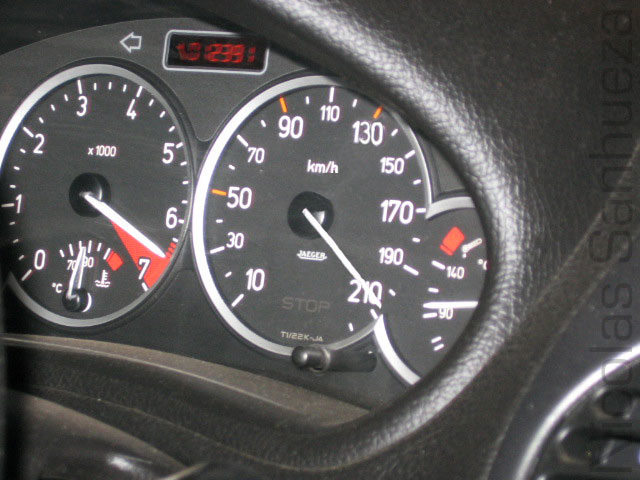In this image, we observe a detailed view of a car's dashboard displaying various gauges. On the left, there is a tachometer, which is marked with numbers from 0 to 7, each increment separated by three small lines. The white pointer is indicating the number 7, situated in the red zone, suggesting high RPM (revolutions per minute). Above the tachometer, the text "x1000" is displayed, indicating that the RPM values should be multiplied by 1000. Positioned above this gauge is a white rectangular display featuring the numbers 0, 1, 2, 3, and 9 in red.

To the right of the tachometer, there is an actual speedometer. This gauge begins at 10 and is marked by a series of small and long lines at intervals representing increments of 10 units, up to 210. The speedometer's long white needle is currently pointing at the 210 mark, suggesting that the car is traveling at 210 units, likely kilometers or miles per hour. Additionally, on the far right side, there is a smaller gauge, with its long white pointer indicating the number 90.

The entire dashboard is encased in a black material typical of most car interiors. Surrounding the gauges is a black dash, characteristic of a car's dashboard. There is also some partially legible text ascending along the right side of the image.